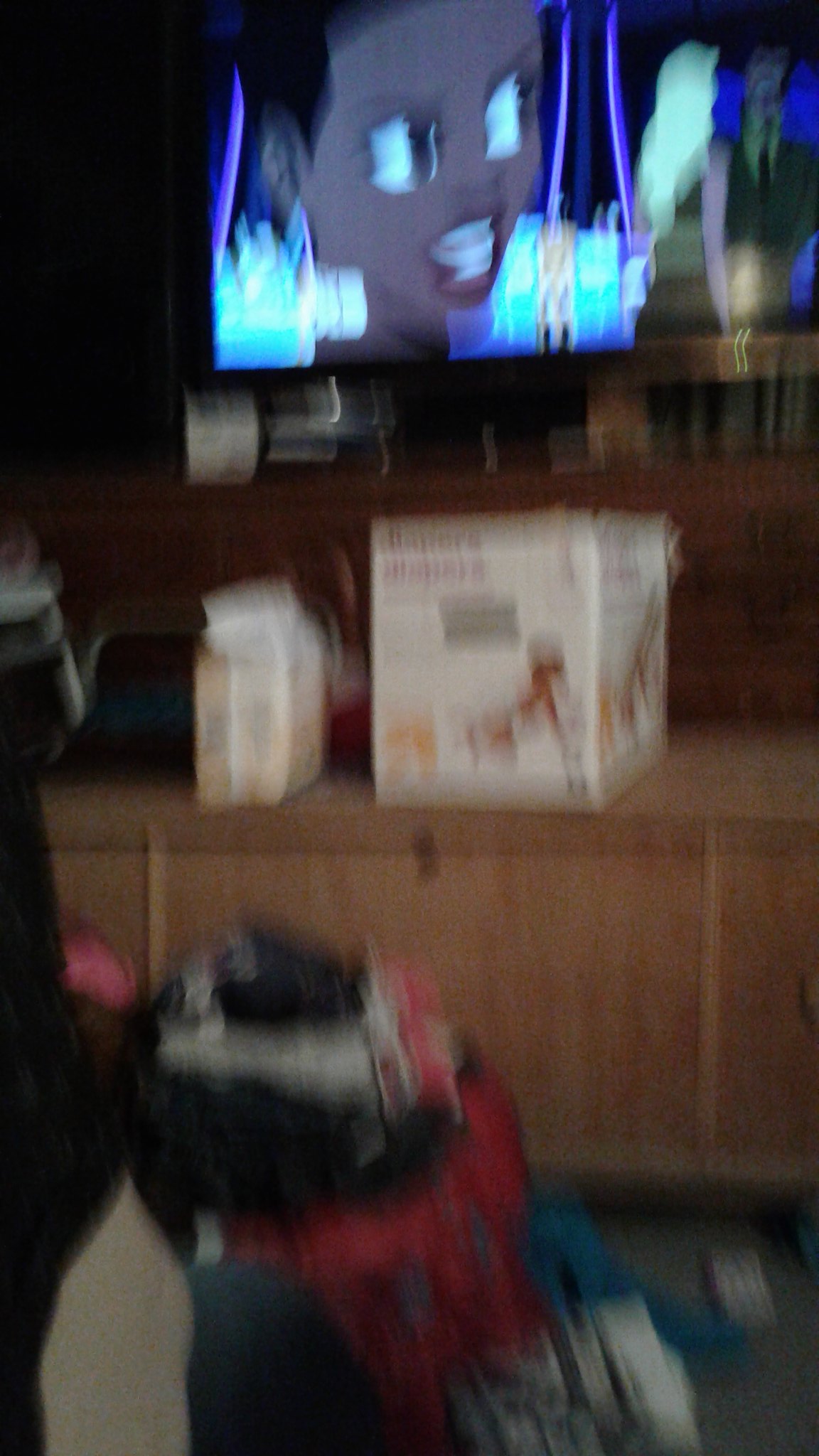A highly blurry image captures the chaotic interior of a living room, scattered with various objects. The central focus is a widescreen TV mounted on the wall, displaying a cartoon with a black actress featuring short hair and red lips speaking to someone off-screen. Below the TV sits a shelf or trunk cluttered with a white box that might be diapers and other miscellaneous items. Numerous clothes and potentially some laundry are strewn across the floor, adding to the clutter. The living room, illuminated with natural light, presents an overall messy appearance. Hanging pots and a counter with cabinets are partially visible in the background, along with a notable red trash can with items spilling out, further contributing to the disarray.